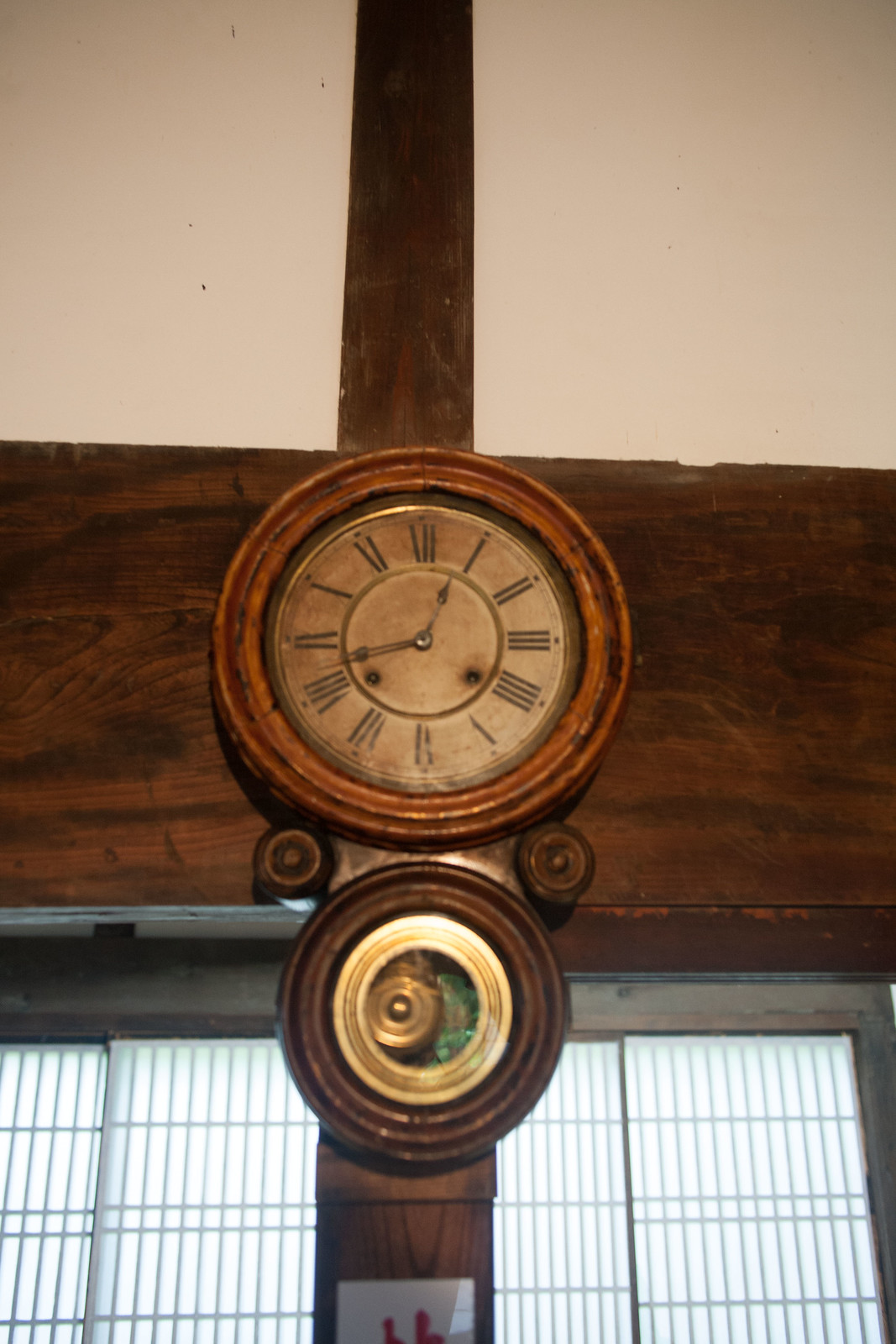The image features an antique clock mounted on a white wall. The wall is characterized by a dark wood beam that extends vertically and then horizontally across the top part of the wall. The clock itself is circular with a light brown wooden frame and a tan interior, featuring black Roman numerals. The clock hands indicate the time is around 12:43 or 12:44. The clock’s face is weathered and shows signs of aging, with two rusted rivets in its metal components. Below the clock is another circular wooden piece with a brass element that appears to be the mechanism housing, resembling the pendulum area of a grandfather clock but lacking the long body. This setup is mounted above what looks like a set of double sliding windows with a white paneling below. The surroundings suggest it is in an institutional building, such as a school, rather than a residential home.